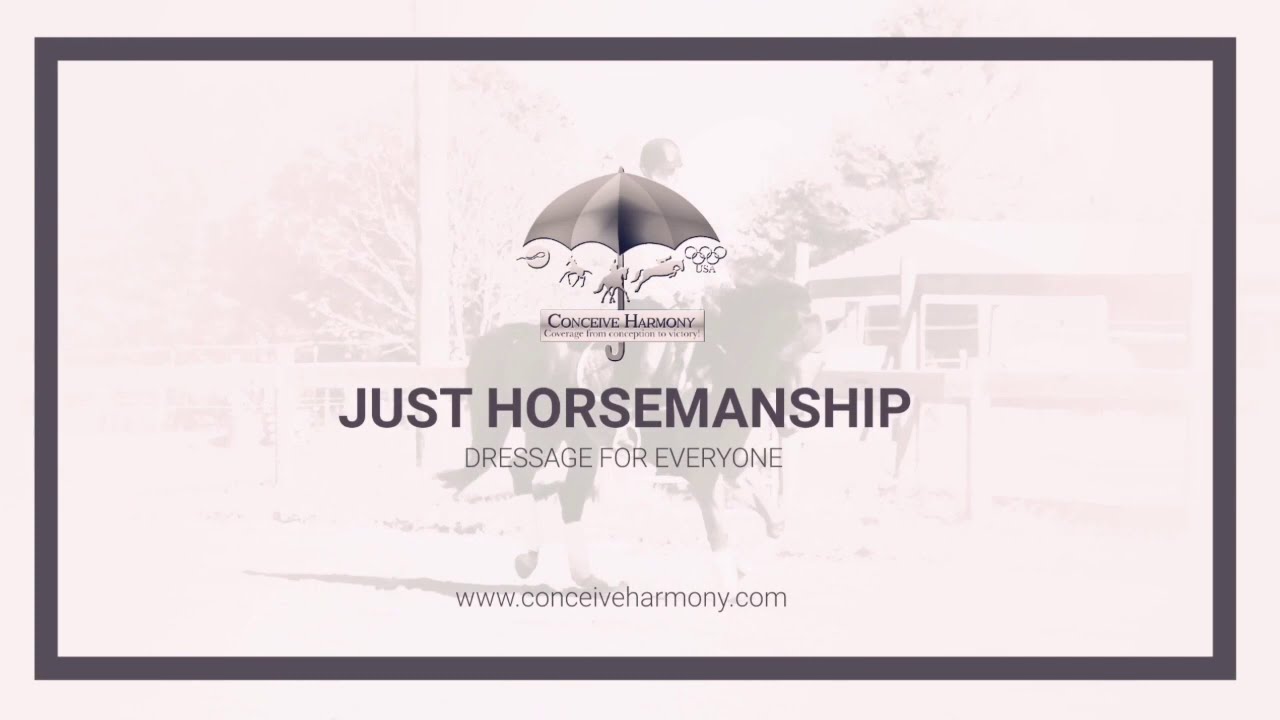The advertisement is a detailed, horizontally-oriented black and white poster for a company called Conceive Harmony. Dominating the center, the bold, light purple text reads "Just Horsemanship" with the slogan "Dressage for Everyone" right below it in uppercase letters. The website address, www.conceiveharmony.com, is neatly positioned underneath. Above "Just Horsemanship," there's an image of a black umbrella, symbolizing coverage and protection, with various illustrations underneath it.

From left to right beneath the umbrella, the images depict a sequence starting with sperm penetrating an egg, followed by a young horse, then a person sitting on a horse, next, a horse and rider leaping over an obstacle, and lastly, the emblematic Olympic rings intertwined with the text "USA." A plaque below the horses reads "Conceive Harmony," reiterating the company's message of "Coverage from Conception to Victory."

The background of the poster features a blurred image of a person riding a horse, who is wearing a helmet, with a building featuring a sloped roof and windows visible in the right background. The entire composition is framed by a darker purple square, which transitions to a light pink background, enhancing the visual appeal of the advertisement.